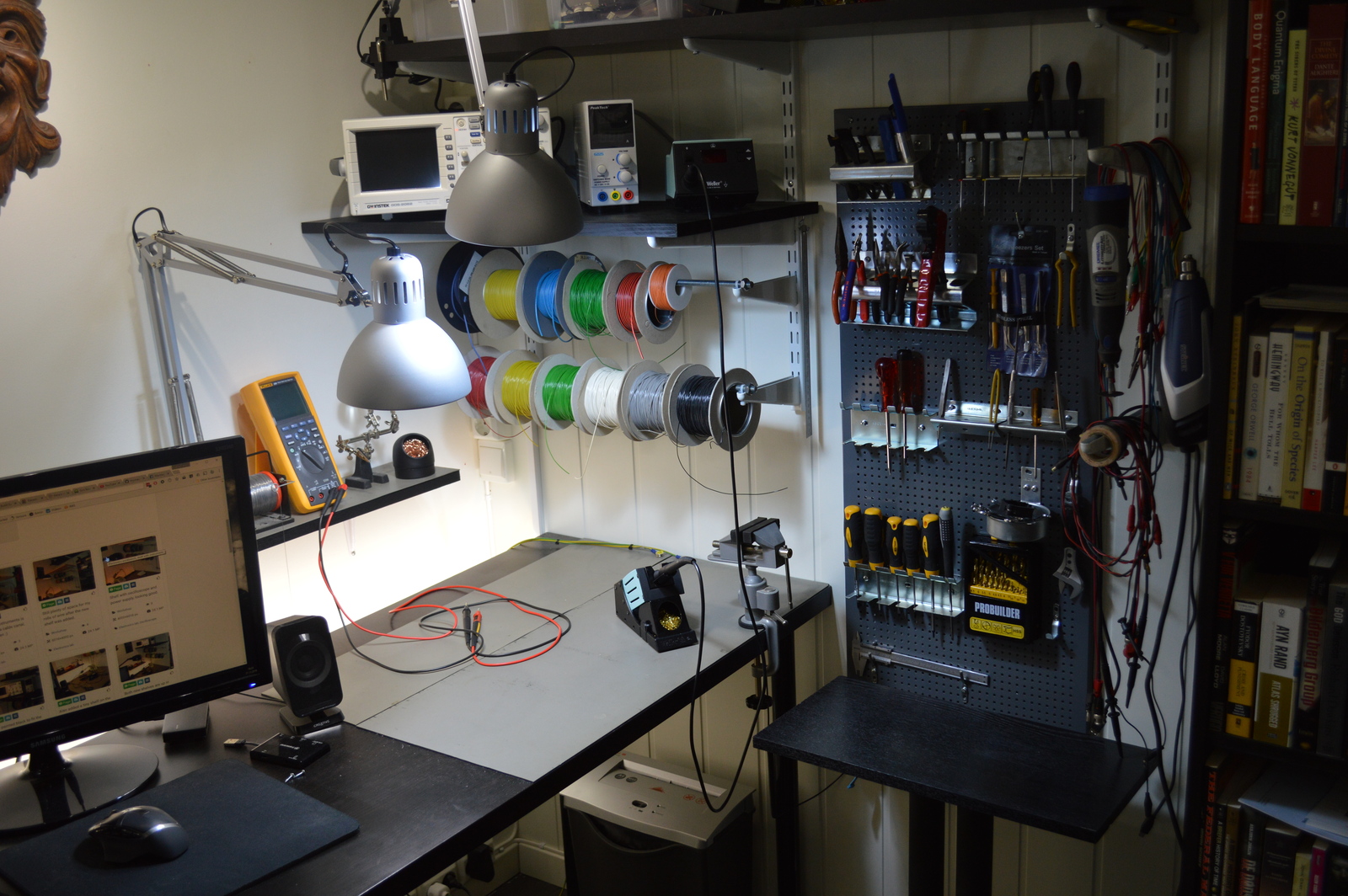This image captures a bustling and organized workshop corner in a room with white walls. The focal point is a desk on the left, equipped with small computer speakers, a mouse pad, a mouse, and an open computer displaying a page with several boxes, possibly relating to shopping or real estate. A white desk lamp points down at the workspace, ensuring ample illumination. Behind the desk, a shelf holds a yellow meter reader and various small tools. Dominating the right side, a wall displays a colorful array of spools with thread or wire in yellow, blue, green, red, orange, white, gray, and black. Above these are multiple monitors. Further to the right, a pegboard is neatly arranged with screwdrivers, screws, and a variety of other tools, alongside hanging drills. Completing the setup, a bookshelf on the far right houses several books. A striking feature of the room is a brown statue of a face mounted on the wall, adding a unique touch to this modern and meticulously organized workspace.